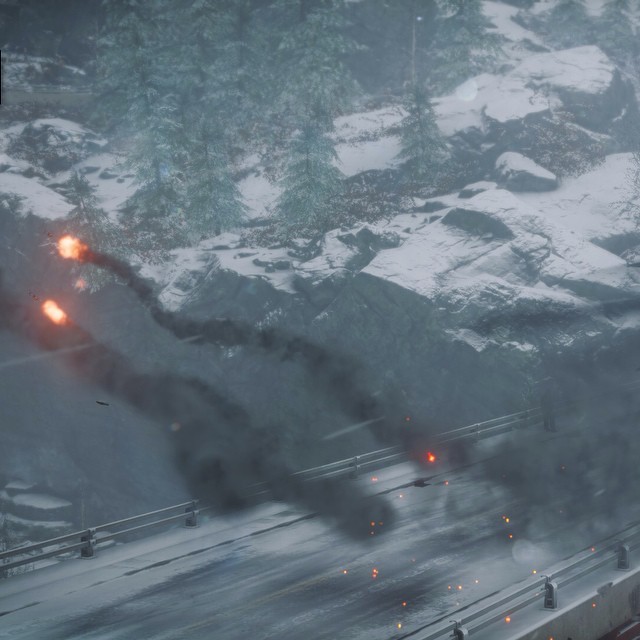This photograph captures a dramatic scene of a mountainous road blanketed in snow and fringed with fir trees, punctuated by the chaos of an explosion. The road, which appears to be part of a bridge, is flanked by safety fences, and the surrounding landscape is dominated by tall rocks and dense clusters of snow-covered fir trees. Thick, dark smoke trails upwards from the site of the explosion, obscuring parts of the horizon. Bright sparks can be seen both in the distance and closer to the left foreground, heightening the sense of imminent danger and heat. The clarity of the photograph leaves it ambiguous whether the white covering is snow or ash from a potential volcanic eruption, adding an element of mystery to the already intense scene.